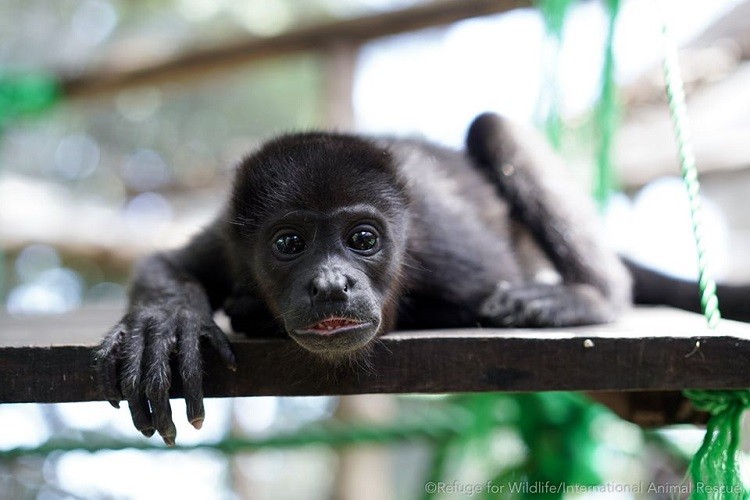In this image, a small black monkey lies on its stomach on a wooden plank, which is suspended by a light green rope visible on the right side of the composition. The monkey's front right hand grasps the edge of the plank, while its rear left leg dangles slightly, with the foot touching the ground and its joints extended. The scene appears to be set in a wildlife rescue facility, as indicated by the text "Refuge for Wildlife / International Animal Rescue" seen in the bottom right corner of the image. The background is highly blurred, showing hints of green foliage and white areas, adding depth without distracting from the subject. The monkey is centered in the frame, looking directly at the camera with a slightly open mouth, displaying hints of pink and red. The color palette of the image primarily includes green, black, gray, white, and brown, emphasizing the natural and rescue-oriented setting.